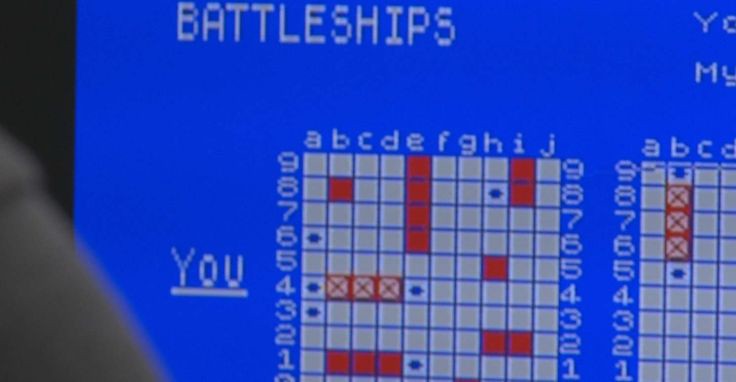The image captures a close-up view of a computer screen displaying the classic game Battleship. The screen has a vintage aesthetic reminiscent of an old computer from the 1980s, akin to a Commodore 64, with a blue background. At the top of the screen, the title "Battleships" is prominently displayed. Below it, a 10x10 grid is visible, labeled with letters A through J along the top and numbers 0 to 9 along the left side.

On the left side of the screen, the word "You" is underlined, indicating the player's grid. This grid contains various markings: red marks presumably showing hits, light gray or white squares signifying undamaged areas, red X's marking missed shots, and blue dots representing unsuccessful guesses. Additionally, there is a partial view of another similar grid, also featuring blue dots and red X's, likely representing the opponent's board.